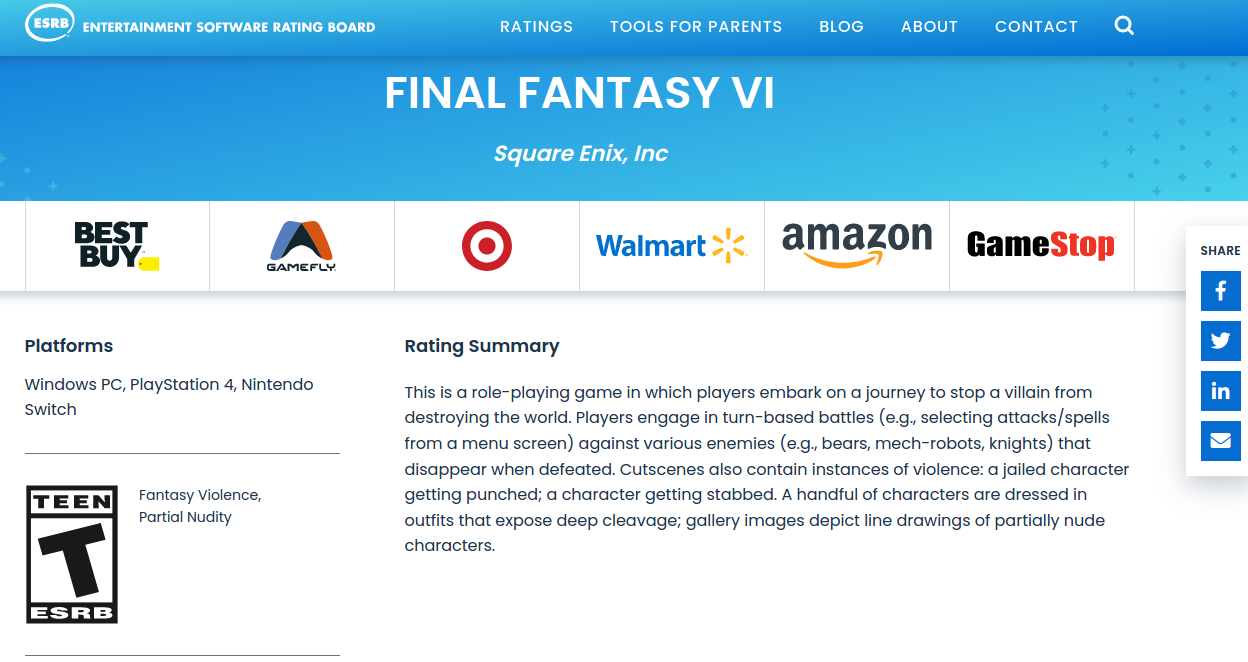This image is a comprehensive screenshot from the Entertainment Software Rating Board (ESRB) website. At the top of the image, the ESRB logo is prominently displayed along with navigation links labeled "Ratings," "Tools for Parents," "Blog," "About," "Contact," and a search icon. The main focus of the page is a detailed rating summary for the game "Final Fantasy VI," developed by Square Enix, Inc.

On the left side, the supported platforms are listed, which include Windows PC, PlayStation 4, and Nintendo Switch. The game is rated T for Teen due to fantasy violence and partial nudity. The rating summary elaborates that "Final Fantasy VI" is a role-playing game (RPG) where players are on a quest to thwart a villain's plans to destroy the world. The gameplay involves turn-based battles where players select attacks and spells from a menu to combat various enemies such as bears, mech robots, and knights, which disappear once defeated. Some cutscenes depict instances of violence, including a character getting punched while jailed and another character being stabbed. Additionally, a few characters wear outfits showing deep cleavage, and gallery images include line drawings of partially nude characters.

To the right are sharing options for Facebook, Twitter, LinkedIn, and email. The image is purely textual and graphical with no photographic elements. There are no depictions of people, animals, plants, flowers, trees, automobiles, or airplanes in the image.